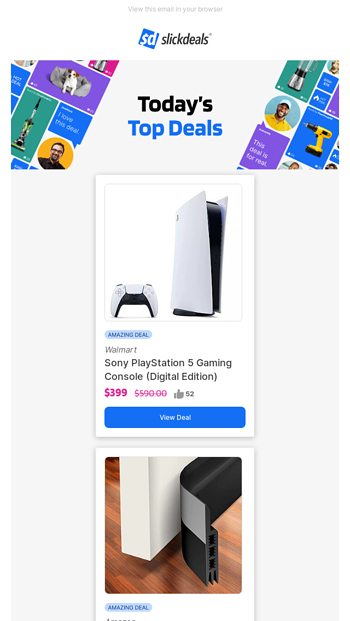In this detailed image, the top portion features a light purple background. Positioned within this area is a small blue box containing a dollar sign and the letter "D," accompanied by text that reads "Slick Deals." Below this, there is a larger segmented box with various sections. 

On the left side of this large box, there is:
- A purple box displaying an image of a dog.
- A green box showcasing a tall, unidentified object.
- A blue box, content unspecified.
- A circular area containing a man's photograph and text stating "Today's Top Deals."

On the right side, there are several smaller boxes each featuring different products, with another circular area displaying a man's photograph.

Dominating the center is a prominent square box featuring the Sony PlayStation 5 Digital Edition gaming console listed at a price of $399 in pink text. Beneath this offer, there is a blue button labeled "View Deal."

Below this main deal, there is another box that includes an image with a white rectangular shape and a small black item beside it. Accompanying this is a blue button labeled "Amazing Deal."